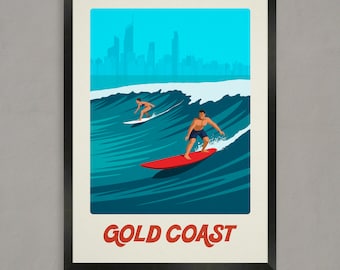The image is a postcard-style framed photo set against a gray background. It features a surfing scene bordered by a white mat and encased in a black frame. At the bottom of the white mat, in large reddish-orange letters, it reads "Gold Coast." The photo shows a vibrant surfing scene with two surfers riding waves under a bright blue sky. The foreground surfer, a man wearing shorts, is on a bright red surfboard, navigating a teal wave with his right leg forward. In the background, a second surfer, possibly female, rides a white surfboard, though the details are more indistinct. The scene is detailed with a cityscape faintly sketched against the horizon, suggesting a distant skyline under clear skies. The curling wave with white froth adds dynamic motion to the illustration, making it a lively depiction of the thrill of surfing on the Gold Coast.